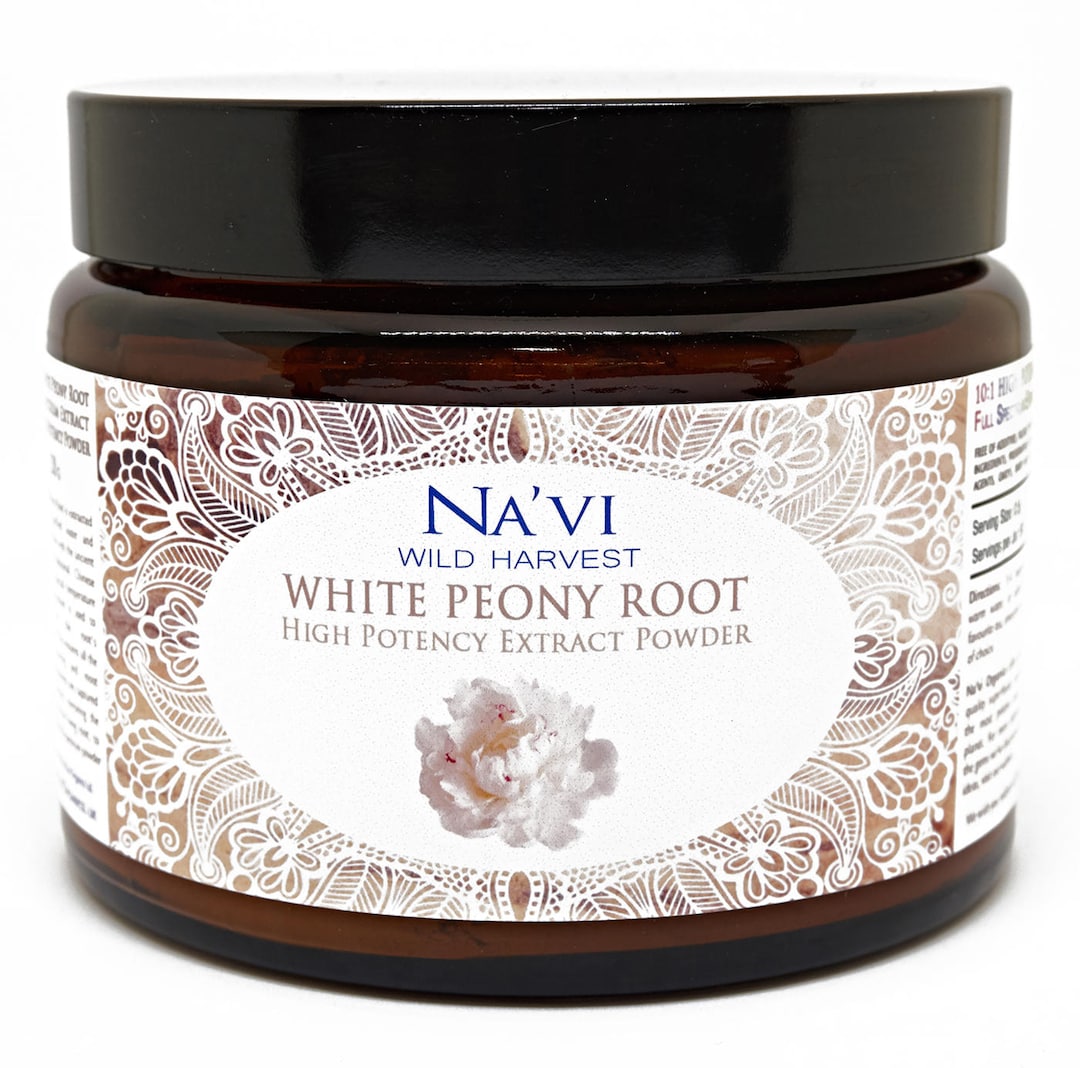The image depicts a wide, squat brown glass jar with a flat black lid. The jar, resembling a dark amber or root beer color, prominently features a label across its front. The label is adorned with an elaborate paisley design in shades of brown and bronze, creating a floral and swirling pattern. Central to the label is a large white oval, within which is a photograph of a white flower. The text within the oval is displayed in two parts: "NAVI Wild Harvest" in blue lettering at the top, and "White Peony Root High Potency Extract Powder" in brown lettering beneath the flower image. The label hints at additional information along its left and right sides, though this text is not fully visible. The jar appears to be a product image, likely for a high potency extract powder supplement.